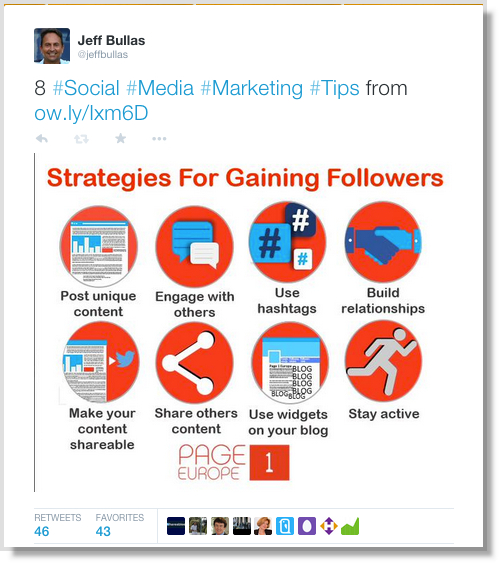*Screenshot of a Tweet by Jeff Bolas (@JeffBolas)*

In this vibrant and eye-catching tweet, Jeff Bolas, a light-skinned man with a tanned complexion and receding hairline, smiles warmly in his profile picture. The tweet contains an informative infographic titled "Strategies for Gaining Followers," which offers several key tips:

1. Post unique content
2. Engage with others
3. Use hashtags
4. Build relationships
5. Make your content shareable
6. Share others' content
7. Use widgets on your blog
8. Stay active

The infographic employs a visually appealing color scheme of red, white, and blue, enhanced by various pictures and icons that make the content more engaging. The tweet has received significant engagement with 46 retweets and 43 favorites, as represented by the corresponding icons displaying the profile pictures of users who interacted with the post.

\*Note: Interactive buttons such as "back," "retweet," "star," and "menu" (the three dots) are also visible, indicating the standard layout of a Twitter interface.